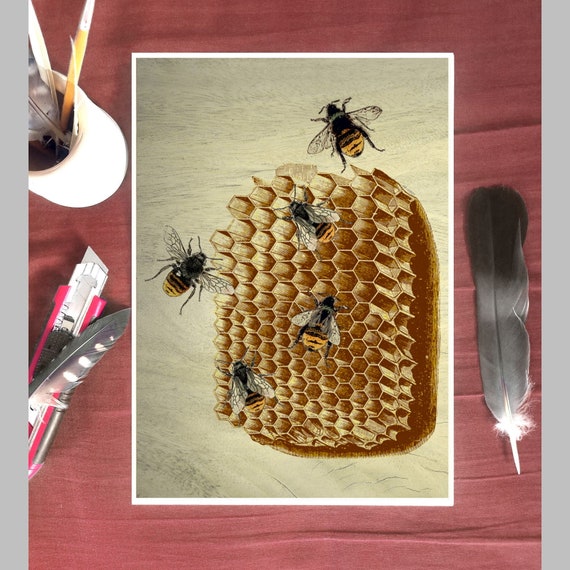The image captures an artfully arranged composition that seems to blend photography with illustration. At its center lies a rectangular depiction of a honeycomb, intricately shaded with darker browns on its right side and bottom, creating a sense of depth. Five bees are meticulously rendered, appearing to hover just above the honeycomb. The honeycomb illustration is set against a cream or tan background, framed by a reddish rectangle resembling a placemat or desk surface with a wood grain-like design.

On the right side of this placemat, a quilled feather transitions from black at the tip to gray and white at the base, adding a naturalistic touch. Alongside it, a white cylindrical pencil holder contains various writing instruments and part of a feather. To the left side, an open pink and silver X-Acto knife lies beneath another feather, which is gray with white highlights. 

The intricate setup, possibly AI-generated due to some incongruous details, gives the impression of a meticulously crafted art scene, combining elements of realism and illustration to create a visually compelling image.